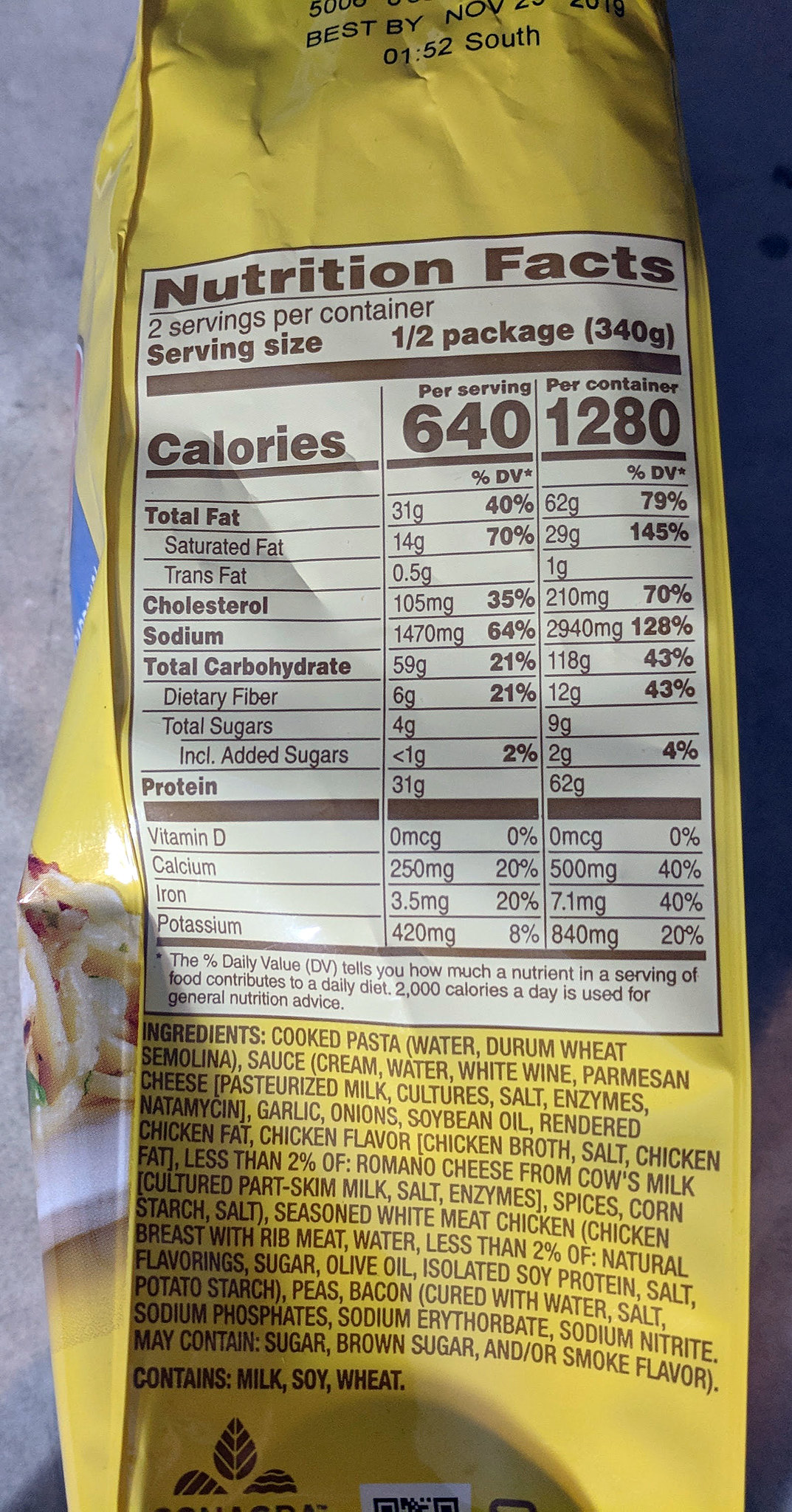The image captures a vertically oriented yellow package taken from a slightly downward angle, offering a partial view of the surrounding environment. To the right, the background exhibits a bluish hue, while to the left, a grayish surface with varied shading and texture, suggesting it might be a countertop, provides context. The zoomed-in perspective focuses on a vibrant yellow package. Prominently featured is a white box detailing nutrition facts, listing the ingredients, serving sizes, and other pertinent information. The package indicates two servings per container, with each serving size being half of the package. A "Best By" date near the top part of the package reads November, ensuring viewers are informed about the product's freshness.